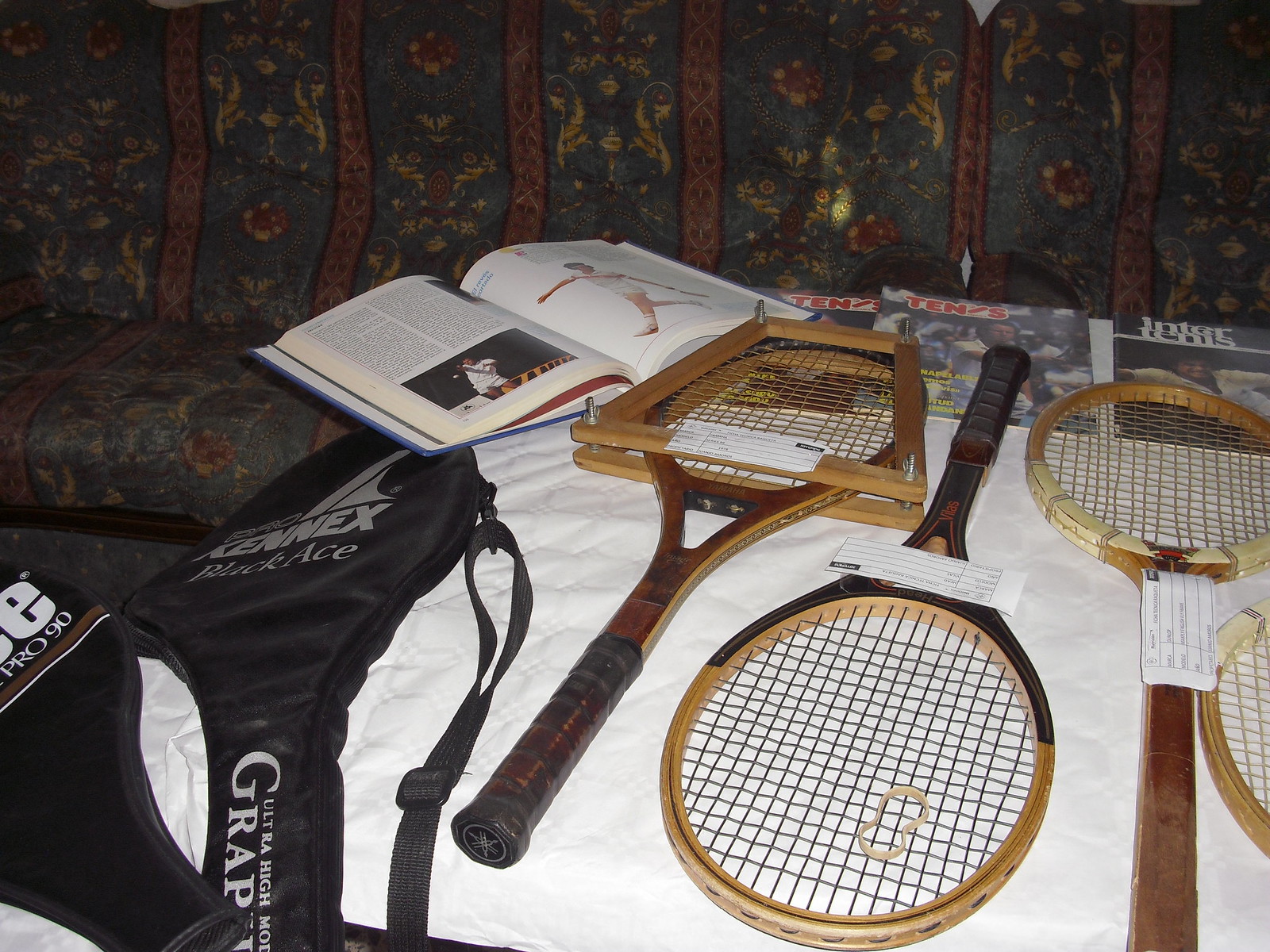The indoor color photograph features a meticulously arranged display of vintage tennis rackets on a table draped with a white cloth, primarily situated to the right of center. The collection includes several wooden rackets, with one prominently featuring an old-fashioned wooden bracket designed to prevent warping. These rackets are alternated with the handles pointing downward and the heads upward, optimizing space on the table. Each racket is labeled as part of a detailed exhibit, possibly within a museum or a dedicated display on tennis history.

The arrangement is complemented by two black form-fitting tennis racket holders placed on the left side of the table. In the background, an open book showcasing photographs and illustrations related to tennis, alongside several magazines with titles such as "Tennis" and "Intertennis," further enriches the display. A blue sofa adorned with a sophisticated gold pattern fabric provides a contrasting backdrop, enhancing the nostalgic ambiance of the scene. Despite being in a somewhat dimly lit room, the subjects are clearly visible, with the elements of the photograph collectively evoking a sense of historical appreciation for the sport of tennis.